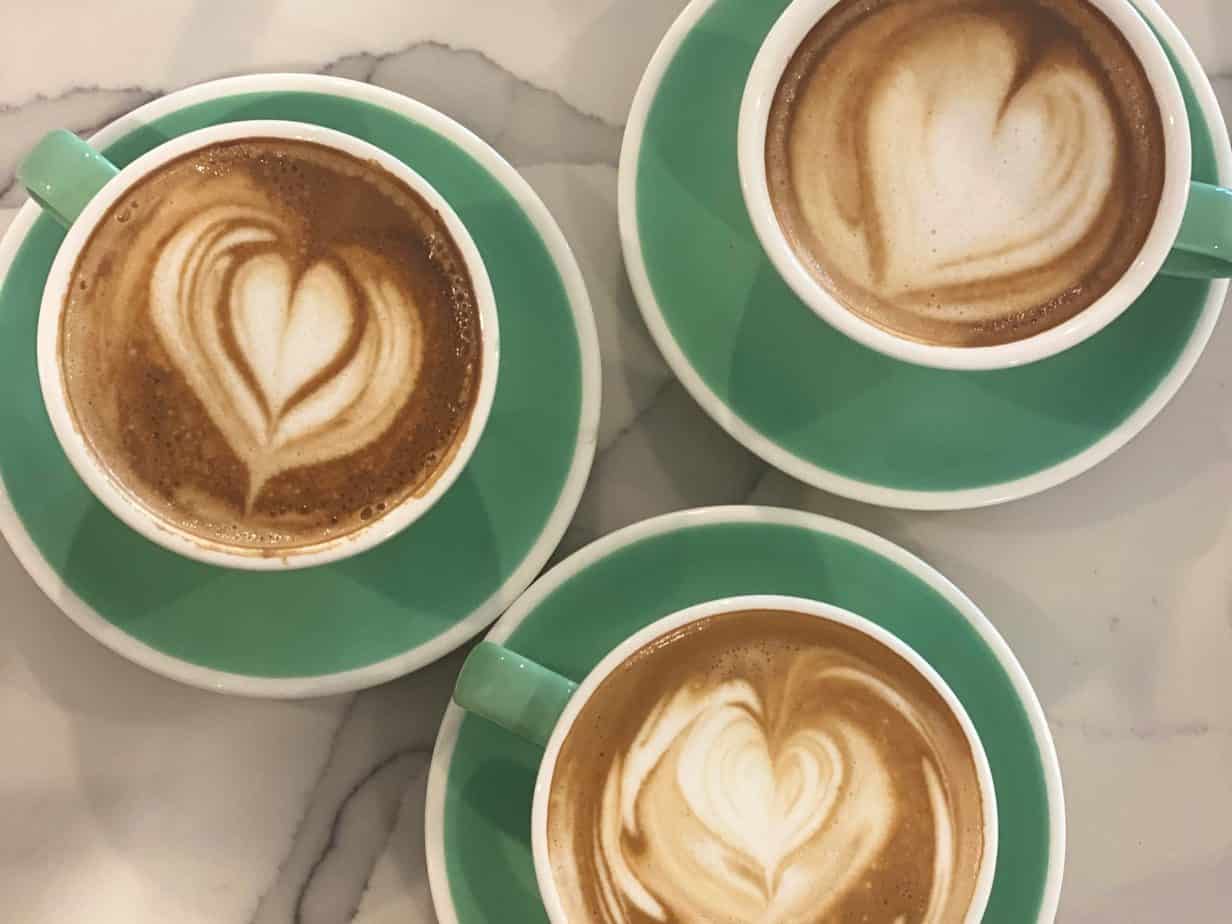The image is a staged, top-down view of three lattes placed on a white marble countertop with black and gray accents. Each latte is served in a green cup with a white rim and matching green saucer. The cups showcase intricate latte art, each with a unique heart design in the milk foam. The upper right cup features a large heart with streaks of brown, but is not as sharply defined. The upper left cup displays a heart bordered by layers resembling petals or leaves, evoking the image of a cut onion. The bottom cup has a lopsided heart, with the right side shorter than the left, and features a brown streak encircling the design. The photograph is square with no border and utilizes artificial lighting to highlight the details of the image.